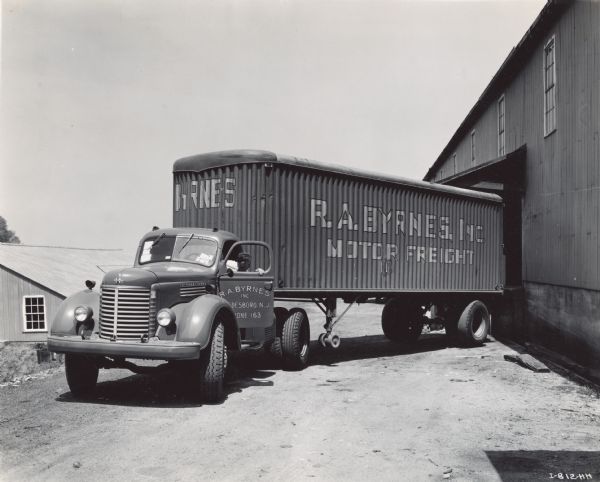A vintage truck is prominently featured in this black and white photograph, its age underscored by the period-specific design and construction. The truck, whose precise color is indiscernible due to the monochrome palette, bears the name "R.A. Burns, Inc." on the cab door, accompanied by an address that is too blurred to decipher. 

The side of the truck prominently displays the text "R.A. Burns and [illegible letters], M.J.T.C.R. Freight" in bold lettering. The truck itself is fashioned from corrugated metal, giving it a rugged, durable appearance. Notably, the cab is equipped with dual sets of tires, enhancing its stability and load-bearing capacity. Twin globe headlights prominently adorn the front of the truck, hinting at the design aesthetics of the era.

Inside the cab, a driver is seated, possibly preparing to navigate the vehicle. The truck is seen in the process of reversing into a large building characterized by wooden siding and multiple second-story windows. The scene is clearly set during daylight hours and takes place outdoors, suggesting a busy industrial or commercial environment.

Overall, the image captures a snapshot of mid-20th-century transportation, with the sturdy truck and attendant signage providing a glimpse into historical freight operations.